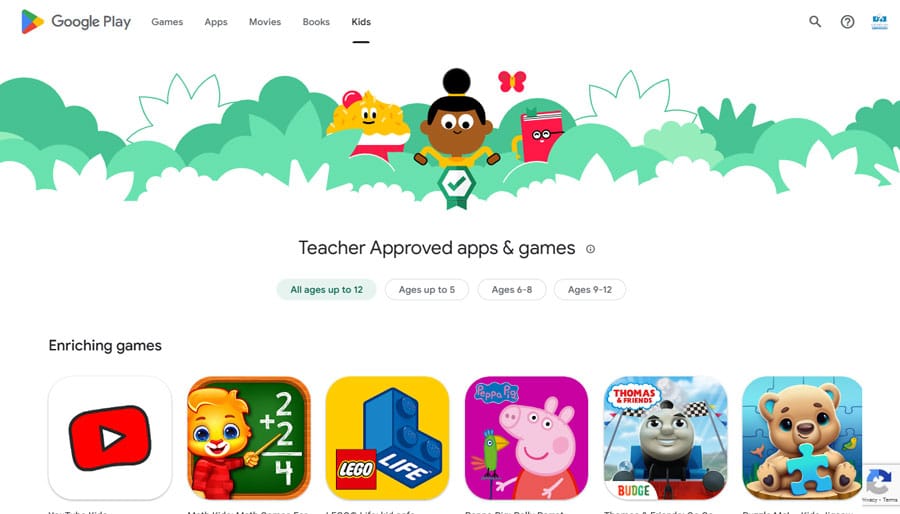The image features a white background with "Google Play" prominently displayed at the top. To the right of "Google Play," there are categories listed: "Games," "Apps," "Movies," "Books," and "Kids." Below this header, the scene transitions into a more whimsical depiction, with illustrated trees and a young Black girl. Accompanying these elements is a book adorned with glasses and a face, suggesting it's anthropomorphized. Alongside the book is a tub of popcorn, similarly animated with eyes, a mouth, and a hat. A butterfly is also seen floating around in this lively tableau.

Beneath this playful imagery, the text reads "Teacher Approved Apps and Games," followed by buttons categorized by age groups: "All Ages up to 12," "Ages up to 5," "Ages 6 to 8," and "Ages 9 to 12." This section is intended to help users find age-appropriate and enriching content.

Further down, the phrase "Enriching Games" is displayed next to an icon resembling the YouTube logo. On the right side of the image, a charming illustration of a cat wearing a red shirt stands in front of a chalkboard. The cat is holding a pointer and gesturing towards the board, which has the simple math equation "2 + 2 = 4" written on it, adding an educational element to the scene.